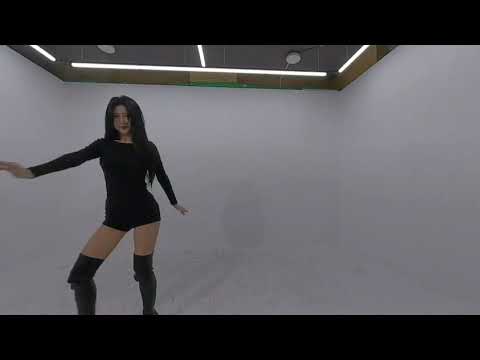In an indoor setting resembling a dance studio with white walls, a woman, possibly of Asian descent, strikes a dynamic pose beneath a ceiling adorned with geometric fluorescent lighting fixtures. She wears a black ensemble consisting of a long-sleeve blouse and very short shorts or a leotard, paired with knee-high or thigh-high boots. Her right arm is extended while her left arm is pulled back, suggesting movement or a dance performance. The background is minimal, highlighting her striking presence against the starkness of the room.